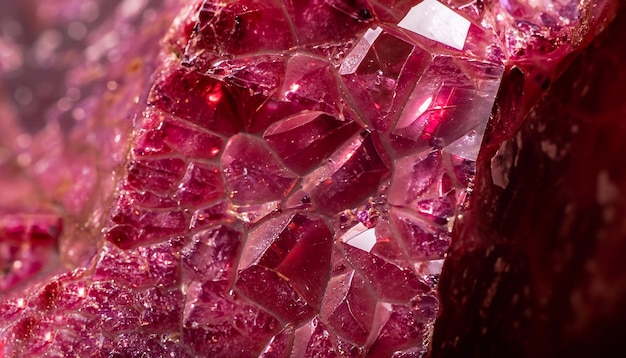This close-up photographic image showcases an intricately detailed piece of purple quartz, likely situated outdoors. The quartz, with its crystalline, glass-like appearance, is shaped rectangularly and is oriented at an angle from the bottom left to the top right. The middle of the quartz features three prominent rectangular protrusions, with natural beveling that resembles precisely cut facets. The image, which serves as an exquisite example of geological beauty, displays a striking combination of purplish and reddish hues, presenting a shiny and jagged surface that hints at its natural formation. The left-hand corner of the image is out of focus but reveals more of the crystalline structure, while the bottom right-hand corner fades into black. The detailed textures and vibrant colors suggest a gem-like quality that could be used for educational purposes, highlighting the enchanting complexity of naturally occurring crystals.